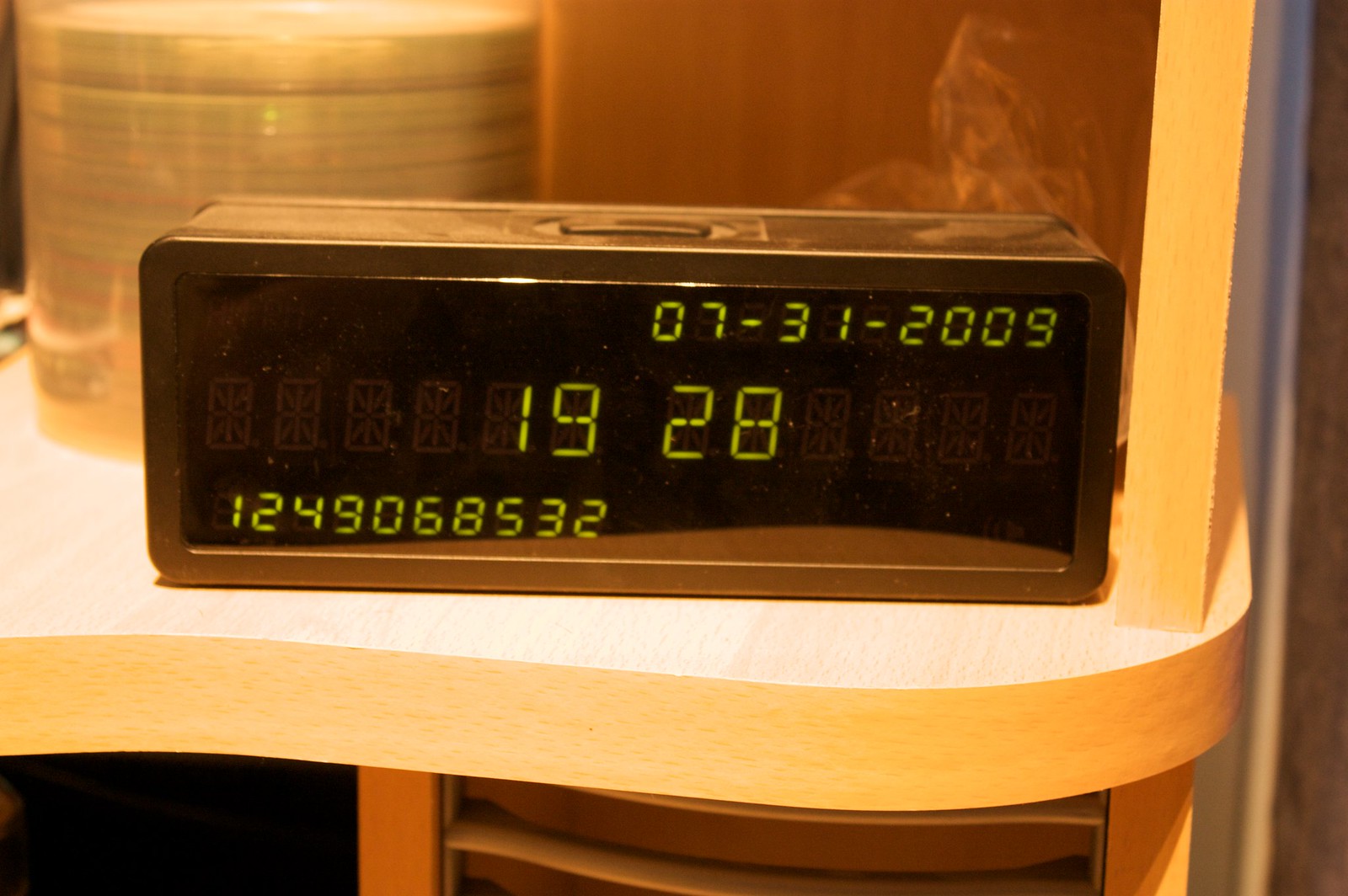A rectangular electronic device, either gray or black, is prominently displayed. Its front panel features a digital display with greenish digits composed of segmented lines, giving it a blocky and uncurved appearance. The device sits on a curved shelf made of light maple wood. Behind it, a blurred cylindrical object is partially visible. A faint, ambiguous haze, possibly smoke, seems to emanate from the device. The digital display shows the date "07-31-2009" at the top, likely representing July 31st, 2009. Below the date, larger digits display "19 28." Another set of digits at the bottom, in a similar size to the date, reads "1249068532."